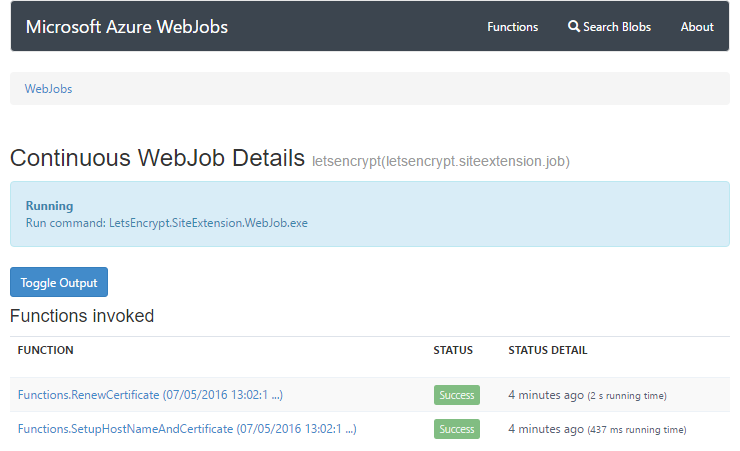The screenshot depicts a webpage from the Microsoft Azure platform, specifically the Web Jobs section. At the top, a dark grey (almost black) navigation bar spans the width of the screenshot. On the left side of this bar, "Microsoft Azure Web Jobs" is written in white. Toward the right side, the bar features the options "Functions," a magnifying glass icon labeled "Search Blobs," and "About," all in white text.

Beneath the dark navigation bar, there's a light grey bar with "Web Jobs" written in blue on the left side. Below this, against a white background, the text "Continuous Web Job Details" appears in black. Additional information is displayed in pale grey, reading "Let's Encrypt [letsencrypt.site.extension.job]."

Further down, a pale blue block contains the word "Running" in bold blue text. Underneath "Running," the following command is presented: "Run Command: letsencrypt.site.extension.webjob.exe."

Near the bottom of the screenshot, there's a small blue rectangle labeled "Toggle Output." Below this button, the section header "Functions Invoked" is written in black against the white background. A pale grey horizontal line separates the header from the subsequent content.

In small black capital letters, the next section begins with the column titles: "FUNCTION," "STATUS," and "STATUS DETAIL." The first row under these titles reads:
- Function: "functions.renewcertificate (07/05/2016 13:02:01)"
- Status: "Success" (indicated in green), 4 minutes ago, with a running time of 2 seconds.

The second row contains:
- Function: "functions.setuphostnameandcertificate" (with a date in brackets)
- Status: "Success" (indicated in green), 4 minutes ago, with a running time of 437 milliseconds.